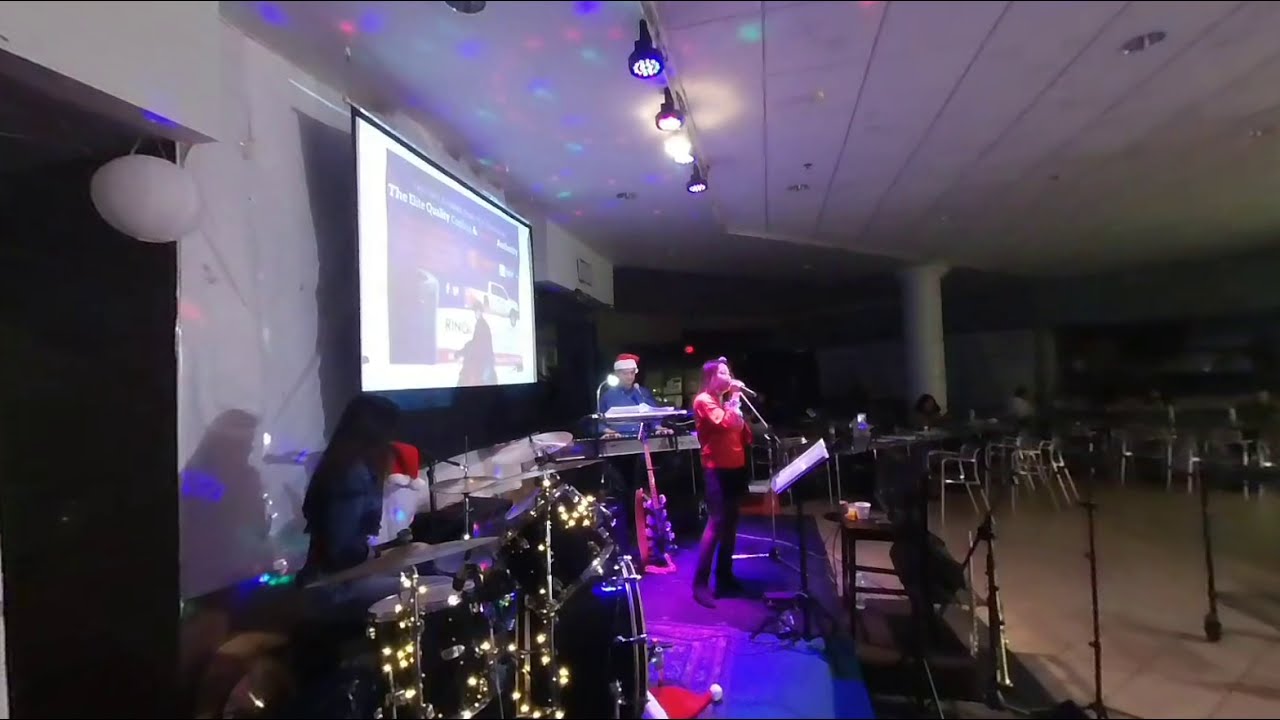In a large room with a white ceiling, a vibrant scene unfolds. A small stage occupies the center, its floor covered in blue. At the forefront, a black, shiny drum set catches the eye. A woman stands confidently behind a microphone stand, her red shirt and jeans striking a contrast. She holds the mic to her mouth as she performs, accompanied by a music stand in front of her. Behind her, a large projector screen displays an advertisement featuring a white truck, creating a backdrop for the performers.

The ensemble includes a drummer in a blue denim jacket and a keyboardist who stands out with a Santa hat and a blue business suit, playing under a lamp shining down on the keyboard. The stage is lit by four spotlights that shine directly on the singer, while a disco ball projects green, red, and blue dots across the ceiling.

Off-stage, the surrounding floor space is open, with chairs and tables neatly arranged on the side, indicating it's a small auditorium setting where a band is playing for an audience. The entire setup suggests a festive and intimate musical performance, blending professional presentation with a touch of holiday spirit.